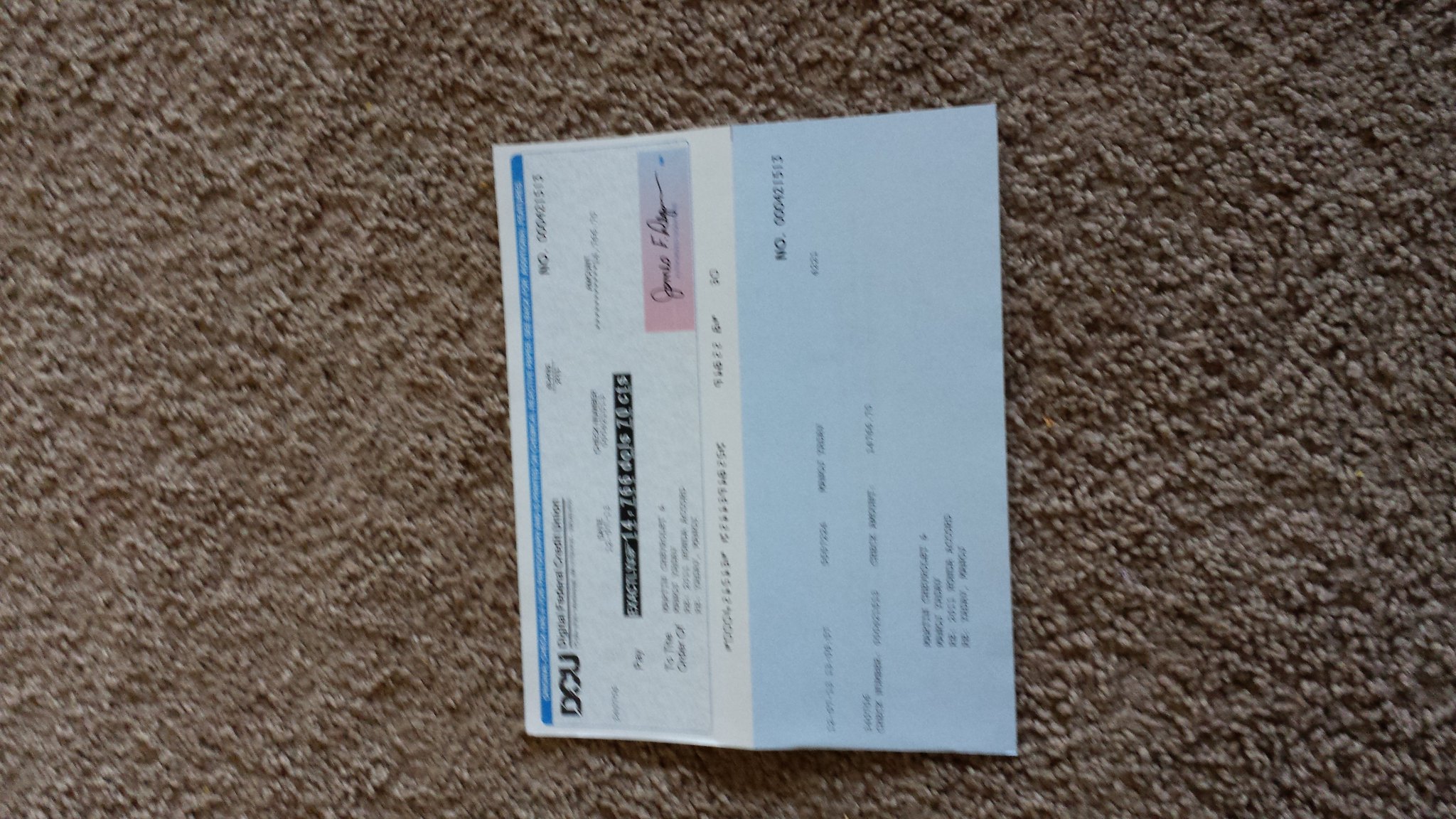The image is a detailed, top-down, landscape-oriented photograph of a bank check lying on a muted brownish-gray carpet. The photograph centrally frames the check, highlighting its placement on the carpet. The check document consists of two main sections: the bank check proper on the left and an attached section of the same size on the right.

The right section of the document is light blue and contains black text, including what appears to be an address. On the left side, the bank check proper features a gradient from purple to blue in the background, with a prominent pinkish signature box located in the bottom right corner, containing a printed, cursive signature in black ink. 

Additionally, a bright blue stripe runs across the top edge of the check, and a black horizontal bar with white text is positioned underneath a logo in the top left corner. The background of the bank check is primarily light blue and white, accented with another long, light blue bar featuring unreadable white text along the left side. The composition and realism of the photograph present the document's intricate details and textures against the modestly textured, older carpet surface.